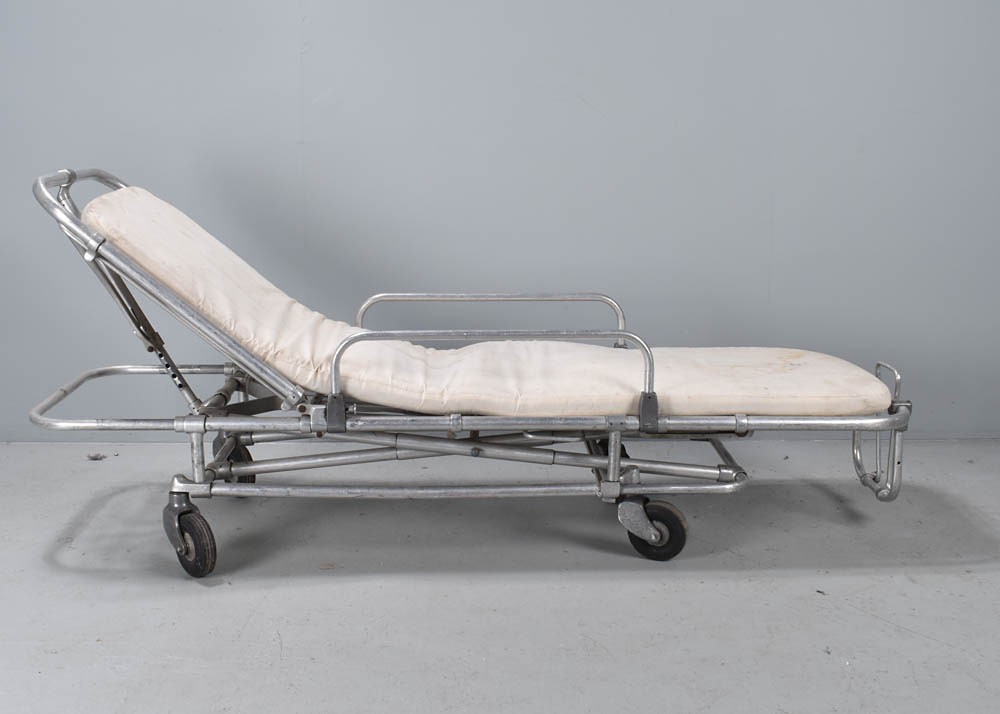The image depicts a worn and aged medical gurney, possibly from a psychiatric asylum or older medical facility. The gurney, centered on the concrete floor with a gray wall backdrop, is predominantly constructed from unpolished silver steel or aluminum. The thin mattress on top of the gurney is heavily discolored, showing yellow and brown stains indicative of long-term use. The gurney's backrest is adjusted to a semi-erect position, angled at approximately 45 degrees towards the left edge of the image. Accompanying the equally worn handrails on the front, back, and sides, there is a noticeable lack of sophistication, hinting at its bygone era. The four black wheels, displaying significant wear, are slightly turned to the right, ready to facilitate maneuverability. Dust and dirt are visible on the gray concrete floor, adding to the overall sense of neglect and abandonment in the stark surroundings.